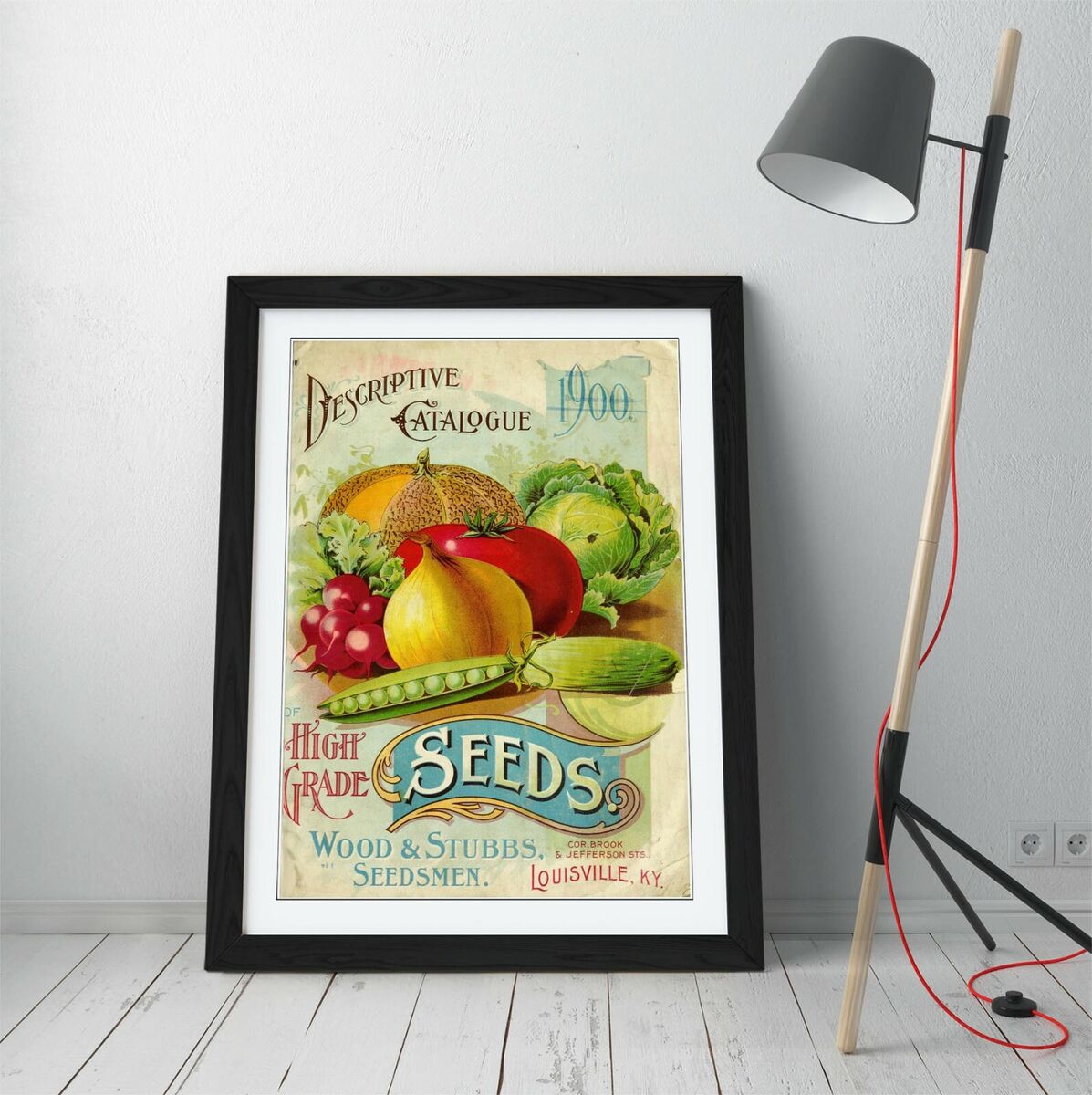This image features a framed poster leaning against a white wall with wood slat flooring. The black-framed poster, bordered by a white mat, displays a vintage-style seed catalog from 1900. The artwork in the center showcases an array of fruits and vegetables, such as cantaloupes, tomatoes, onions, peas in the pod, and lettuce. The text on the poster reads "Descriptive Catalog 1900" at the top, followed by "High Grade Seeds, Wood and Stubs, Seedsmen" underneath. Further down or to the side, it lists "Coor, Brock and Jefferson, Louisville, Kentucky," likely indicating the seed company's location. To the right of the frame stands a lamp with a black lampshade on a narrow stick-like holder, accentuated by a red cord, ready to illuminate the scene. This depiction suggests the poster is a reproduction of a seed catalog cover, intended for sale, possibly online or in a catalog, presented as it might look when framed and displayed in a home.